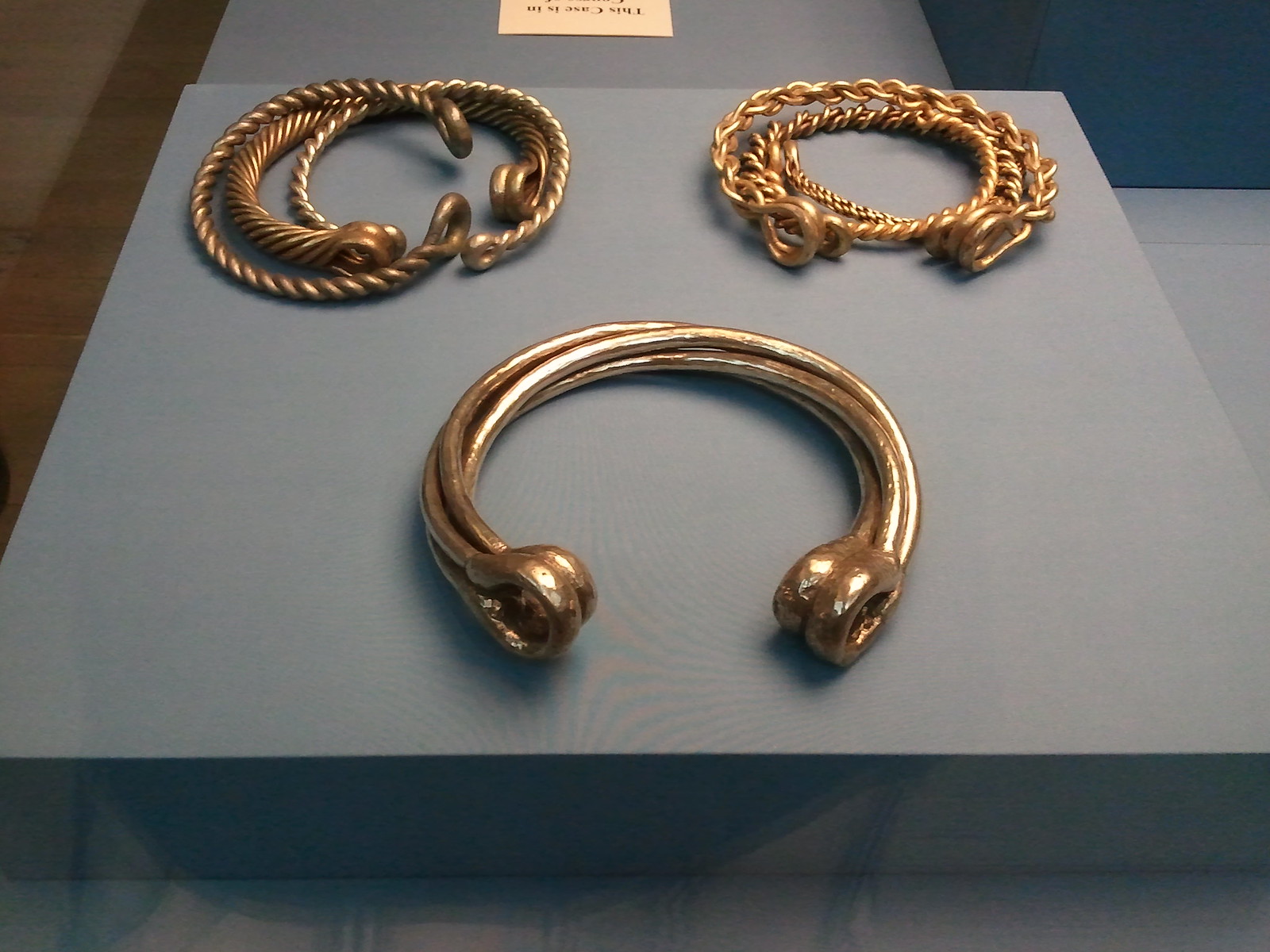This photograph captures an assortment of intricate jewelry, elegantly arranged on a gray display block within a glass case, as suggested by the faint reflection at the bottom of the image. The pieces exhibit a classic vintage aesthetic, crafted from what seem to be gold and bronze metals, possibly even silver. 

The display is organized into three distinct sections. The section located at the bottom closest to the viewer features simple, rounded open bracelets that taper into slightly thicker ends with small hooks, suggesting they might be designed to hold additional charms or embellishments. 

In the top left section, more elaborate pieces are on display, designed to resemble coiled ropes, with a braided texture highlighting the artistry of the metalwork. They appear as though smaller, twisted metal strands are intricately woven together, giving a sense of both strength and finesse.

The top right section showcases jewelry that appears to be chains linked together, displaying a sophisticated interlocking design. One notable piece among these seems formed from multiple wires braided together to create a double loop, emphasizing both beauty and durability.

Overall, the collection consists of what looks like a variety of bracelets, each meticulously crafted, hinting at both historical significance and timeless elegance.